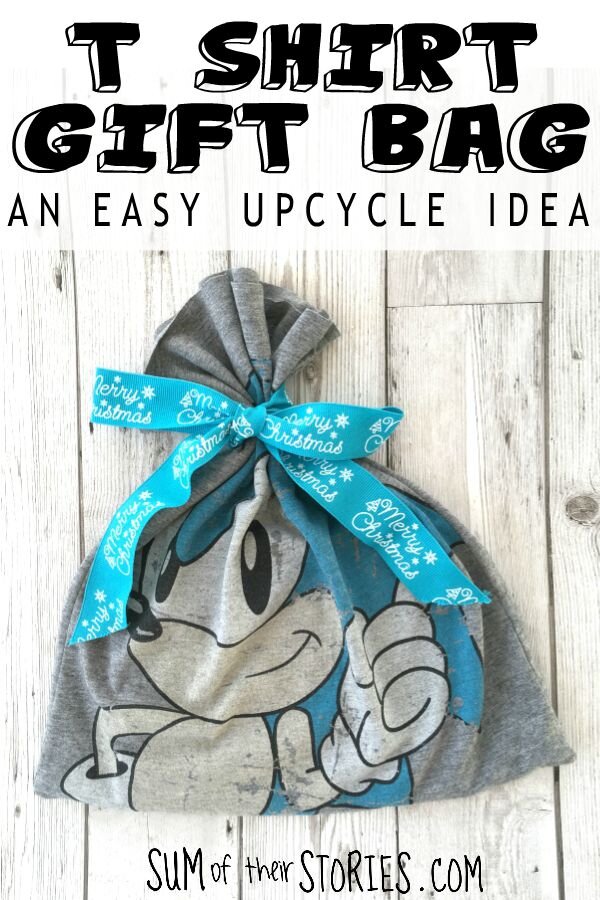In this picture, we see an advertisement at the top that reads "T-shirt Gift Bag" in bold block letters with a white edge. Below, it says "An Easy Upcycle Idea." The central image features a grey T-shirt that has been creatively upcycled into a gift bag. This T-shirt displays a vibrant image of Sonic the Hedgehog, showcasing Sonic's iconic blue hair and raised fist. The T-shirt is secured with a neat blue ribbon, adorned with the words "Merry Christmas" in white lettering. The T-shirt bag is placed on a grayish wooden platform, and towards the bottom of the image, we notice a reference to a website: someoftheirstories.com.